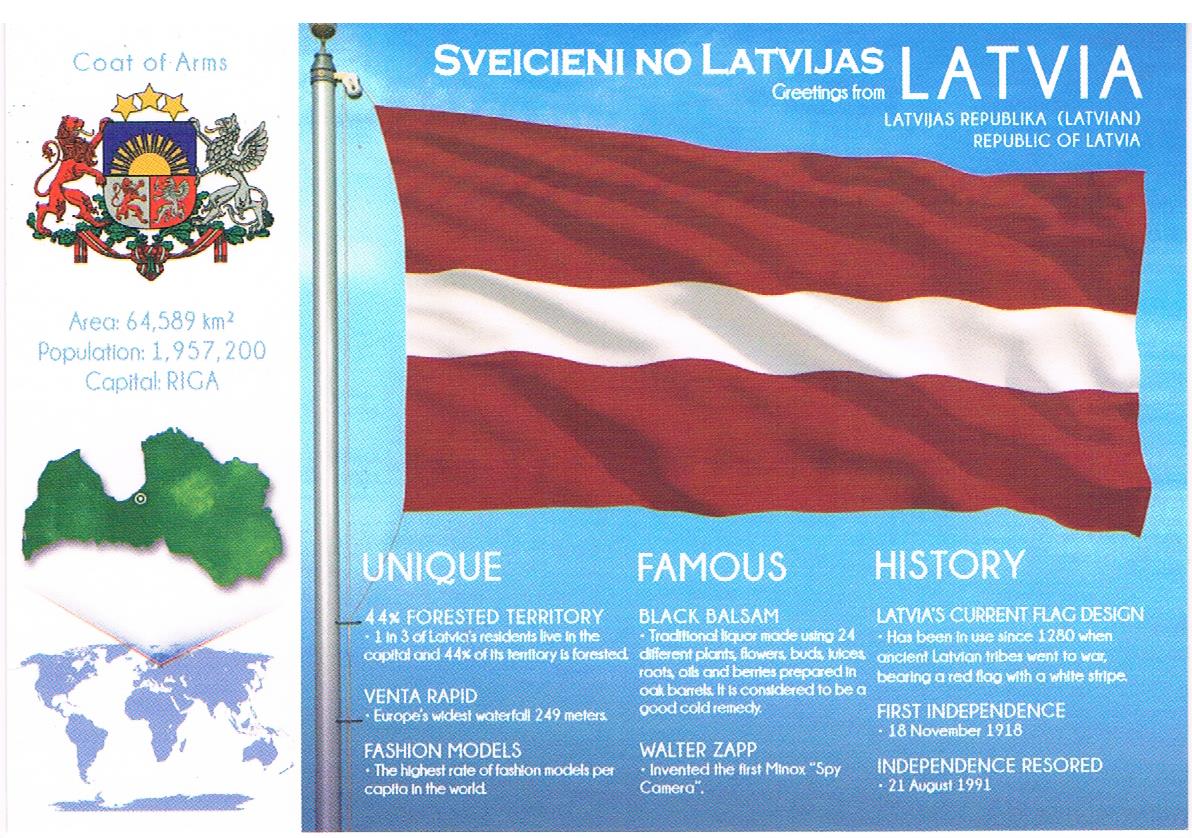The image is a detailed infographic about Latvia on a blue background. Dominating the right three-fourths of the graphic, the Latvian flag with its horizontal red-white-red stripes stands prominently. Above the flag, white text reads "SVEICIENI NO LATVIJAS" (Greetings from Latvia) and "Republic of Latvia." The content is categorized into three sections: 

1. **Unique**: Highlighting that Latvia boasts the highest rate of fashion models per capita in the world, with 44% of its territory forested.
2. **Famous**: Mentioning Walter Zapp, inventor of the first Minox spy camera, and the presence of Europe's widest waterfall, Venta Rapid.
3. **History**: Noting Latvia's first independence in 1918 and the restoration of independence in August 1991.

The left side of the graphic features a vertical white strip with Latvia's coat of arms and a detailed map indicating Latvia's location. Furthermore, it provides essential stats: the area of 64,589 km², a population of 1,957,200, and its capital city, Riga.